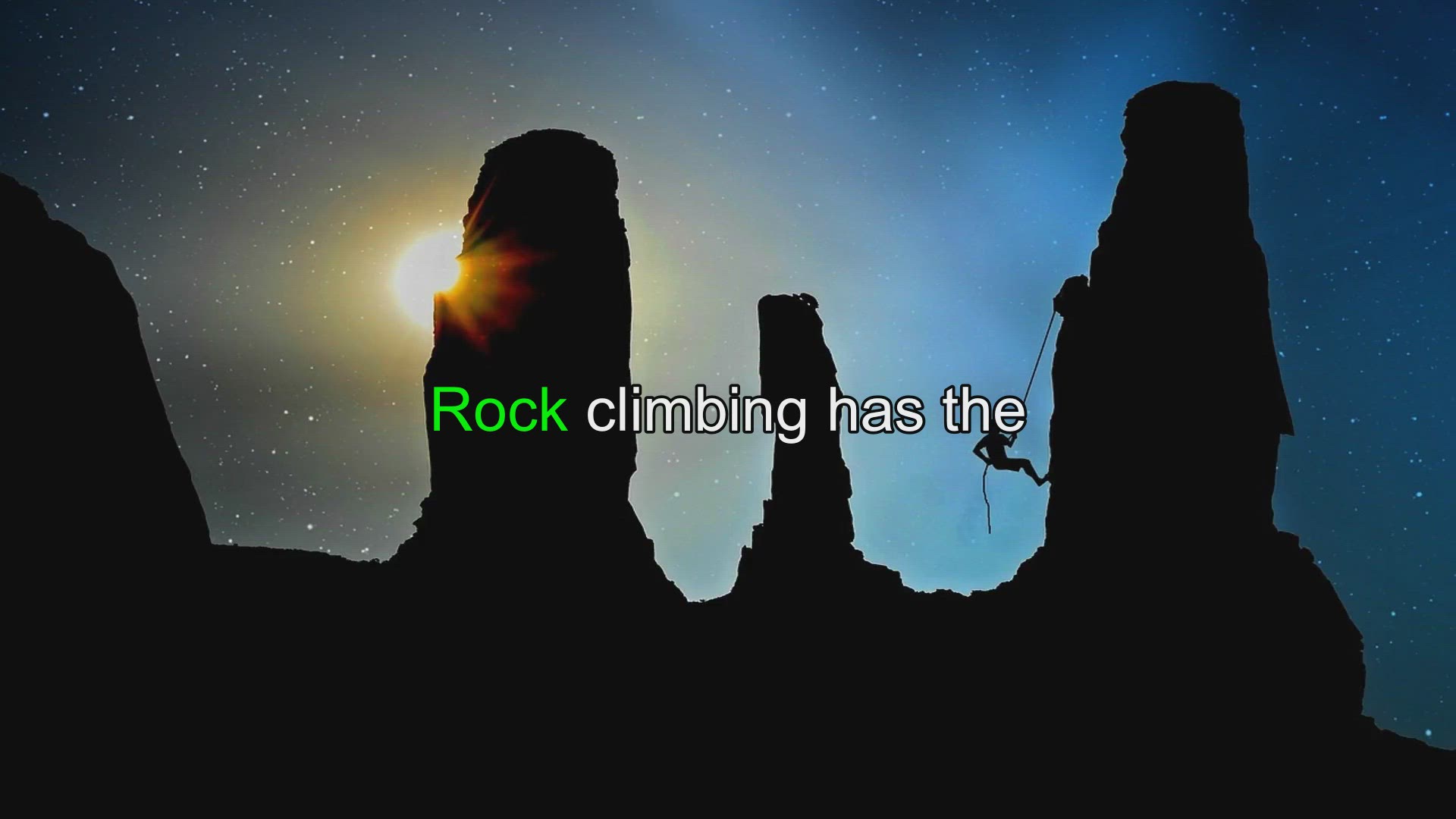The image, reminiscent of a postcard or poster, depicts a striking nighttime scene of four silhouetted rock formations against a starry sky. The formations, which create an undulating pattern resembling a 'W,' stretch horizontally from left to right. The leftmost and rightmost peaks are the tallest with the rightmost one being the highest and featuring a climber scaling its face with ropes. A dark blue sky, gradually lightening to the right, serves as the backdrop, dotted with stars. Intriguingly, a large moon hovers near the left side, partially obscured by the rock formations, casting its rays towards the upper left of the image. Adding to the mysterious ambiance, there appears to be the sun peeking halfway out from behind the leftmost rock formation. The words "ROCK" in green and "CLIMBING" in white are prominently displayed across the center, adding a bold textual dimension to the visual composition.